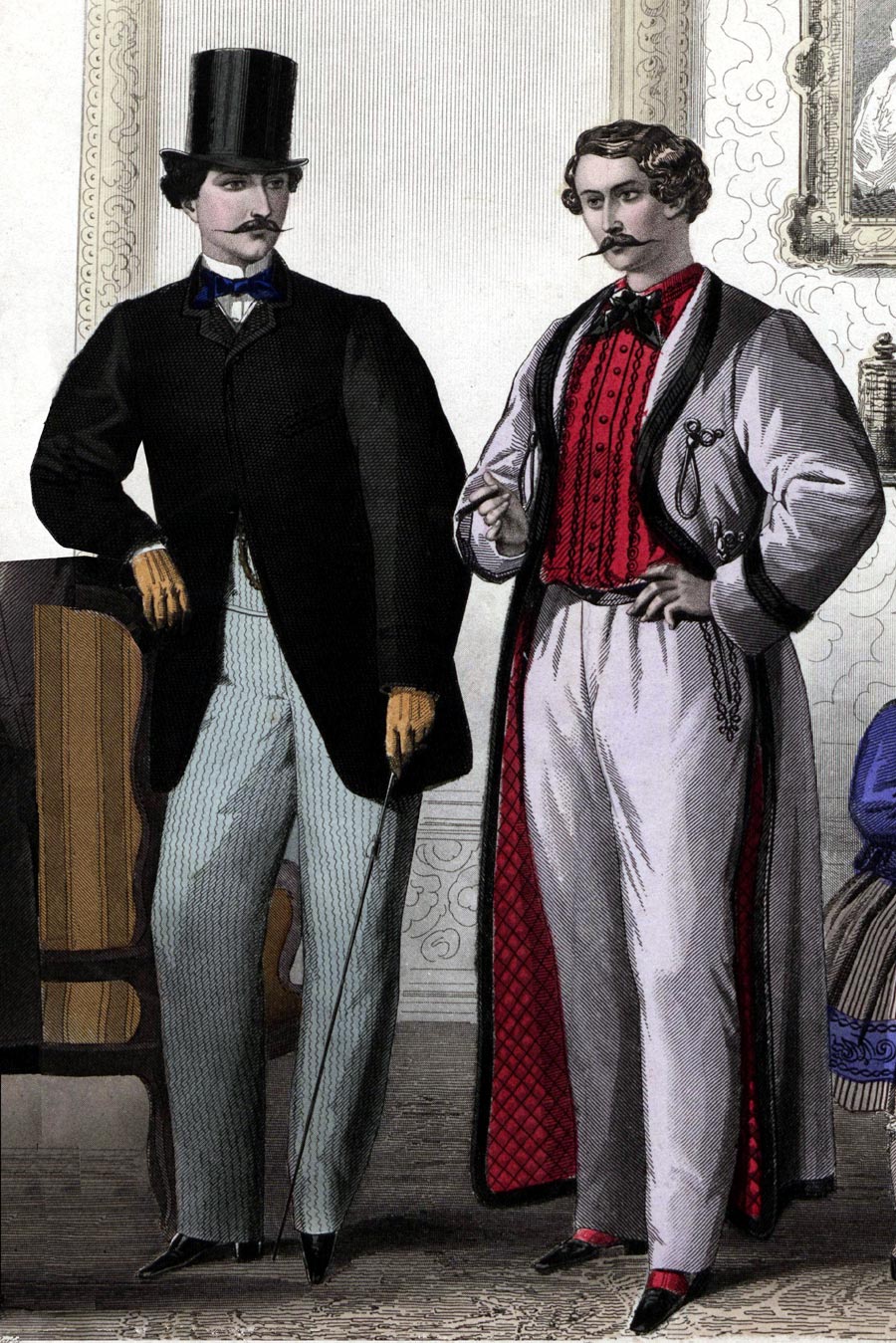This painting depicts an old-timey setting featuring two white men dressed in 19th-century fashion, standing against a plain white background. The man on the left is distinguished by his tall black top hat, from beneath which bushy hair protrudes. He sports a long, curled mustache, a white shirt with a black bowtie, and a large black overcoat. His hands, covered by yellow gloves, grasp a black cane. He completes his ensemble with striped pants and polished black shoes. Beside him, the second gentleman wears a long, white robe-like jacket over a red shirt, also adorned with a black bowtie. He, too, has curly, bushy hair paired with a handlebar mustache but does not wear a hat. His lighter-colored pants, possibly light gray, complement his outfit, and his black shoes feature a distinctive red accent across the upper part. The men appear to be engaged in conversation, capturing a moment of casual interaction from a bygone era.